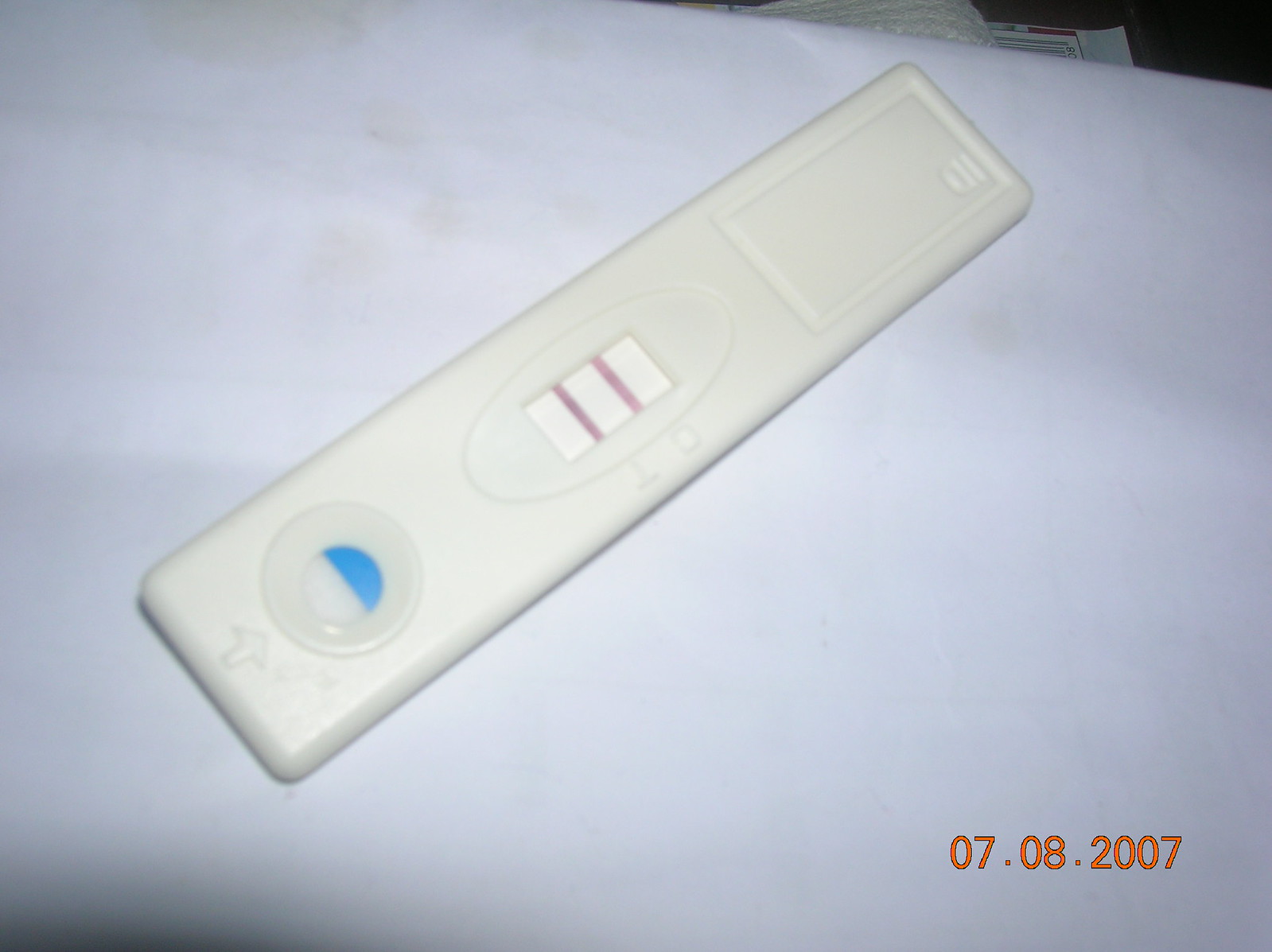The image depicts a detailed and organized scene featuring a medical test kit. In the lower right corner, labeled in bold orange text, is the date "07.08.2007". The kit rests on a thin white placemat that appears slightly worn, with subtle yellow or dark beige stains visible in the upper left corner. 

At the center, there is a long rectangular test strip, approximately seven to eight inches in length and about two inches high. To the left of this test strip, a tiny arrow points towards a circular indicator divided into two halves: one blue and one white.

Moving down the image, another component catches the eye - a longer, sideways oval frame enclosing a white rectangle marked with two straight, vertical pink lines. Adjacent to this, a regular white rectangle matching the color of the test kit is seen.

The overall impression is that of a diagnostic tool, potentially a blood test or a pregnancy test, designed to indicate results through a color-coded system involving blue and pink hues.